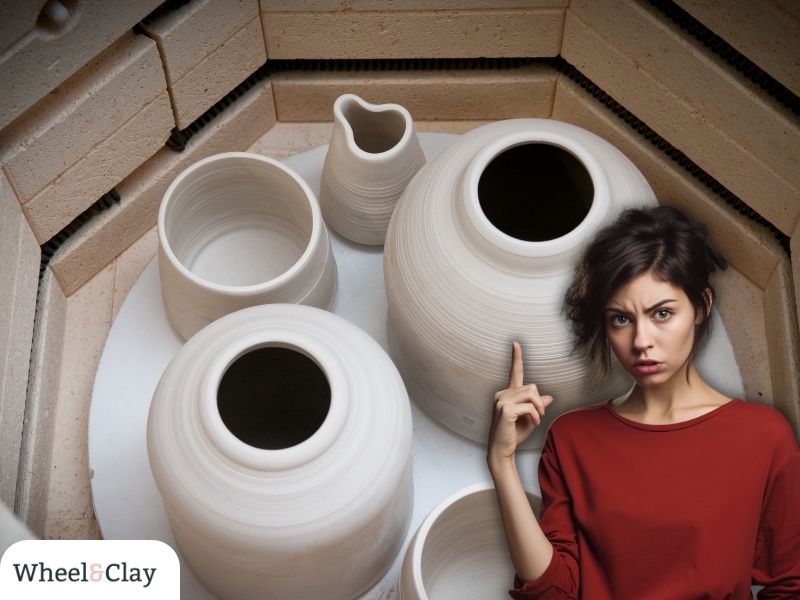In the bottom right corner of the picture, a woman with her hair tied back is seen pointing upward with her right hand. She is wearing a red long-sleeve shirt and has a dark brown hair. Her expression is one of anger and concern. Behind her, there is a collection of ceramic pots placed within a hexagonal brick structure. The bricks are light brown, and the pots, which are light gray in color, have a clay-like appearance. One of the pots is noticeably warped, indicating a possible flaw, while the others appear to be intact and well-crafted. At the bottom left of the image, text reads, "Wheel of Clay."